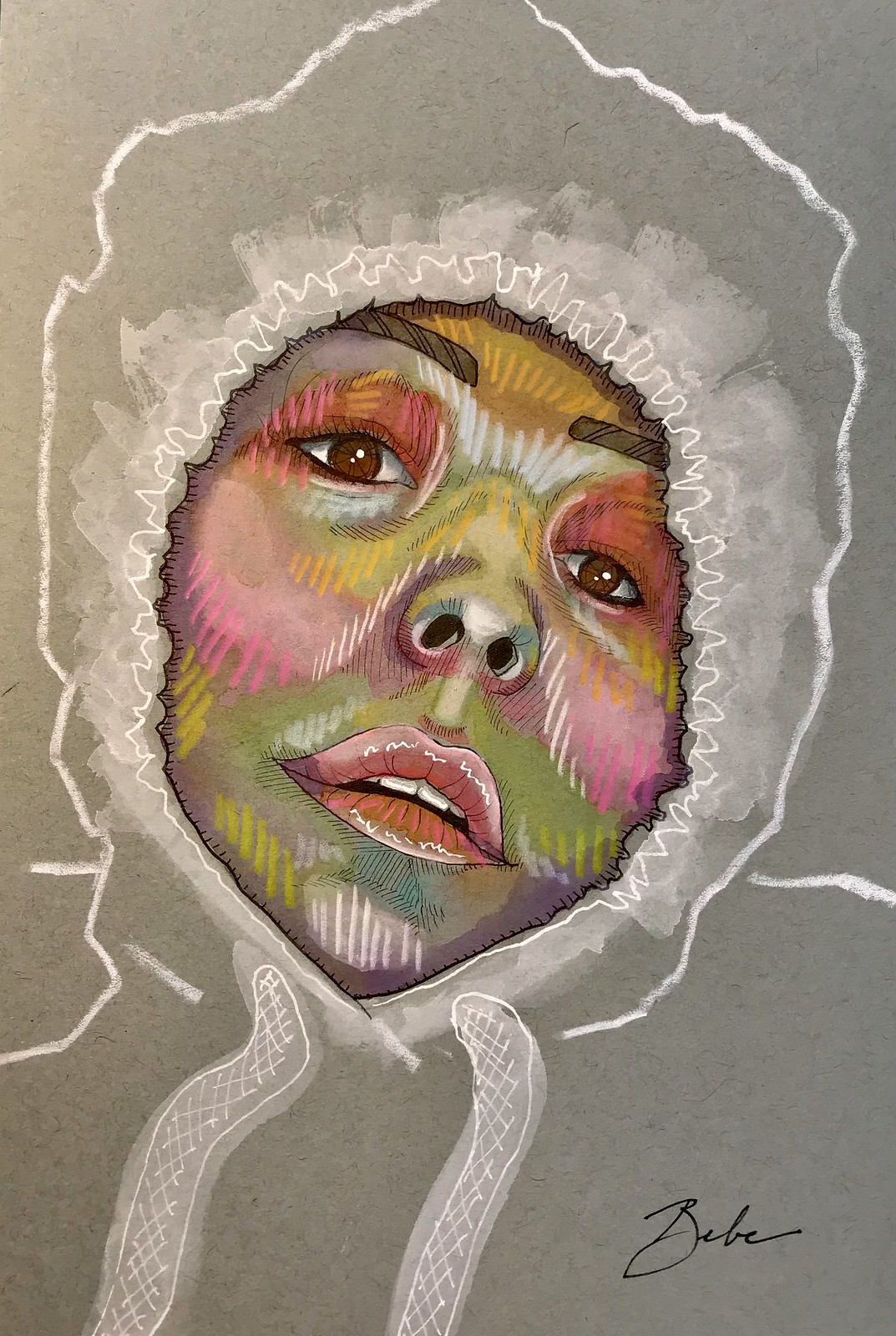This vibrant illustration captures the striking visage of a woman rendered in an artistic painting style. Her face is a kaleidoscope of colors, with pink and green tones blending harmoniously across her skin. Her full, luscious lips are painted a bold red, adding a focal point to the composition. Emerging from a textured gray backdrop, her face is outlined and surrounded by a soft, white halo that accentuates her features. In the bottom right-hand corner, the artist's signature, "Bebe," is elegantly inscribed, adding a personal touch to this captivating piece of art.